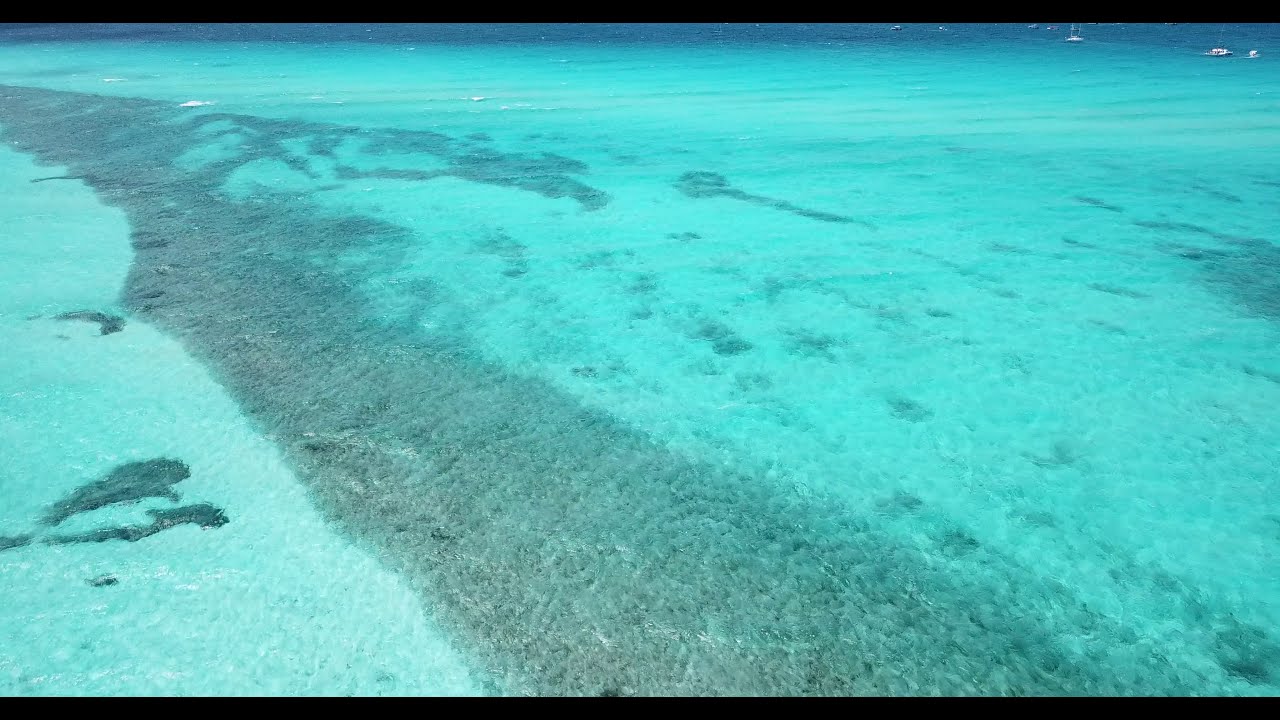This captivating image showcases a vibrant, turquoise section of the ocean, rendered in stunning clarity and depth. The foreground is dominated by translucent, neon-green water, hinting at its shallowness, with visible mounds of dirt and suspected underwater features like rocks or coral reefs scattered throughout. As your eyes move upwards, the hue deepens to a darker blue, particularly pronounced at the top of the image. The upper right-hand corner reveals a cluster of tiny white boats, about six or seven, dotting the otherwise empty expanse of water. The overall scene is framed in a rectangular, horizontal format with thin black stripes running along the top and bottom edges. The detailed and almost mesmerizing contrast in water color—from the light, almost teal green to the deep ocean blue—enhances the tranquil yet dynamic quality of this underwater vista.